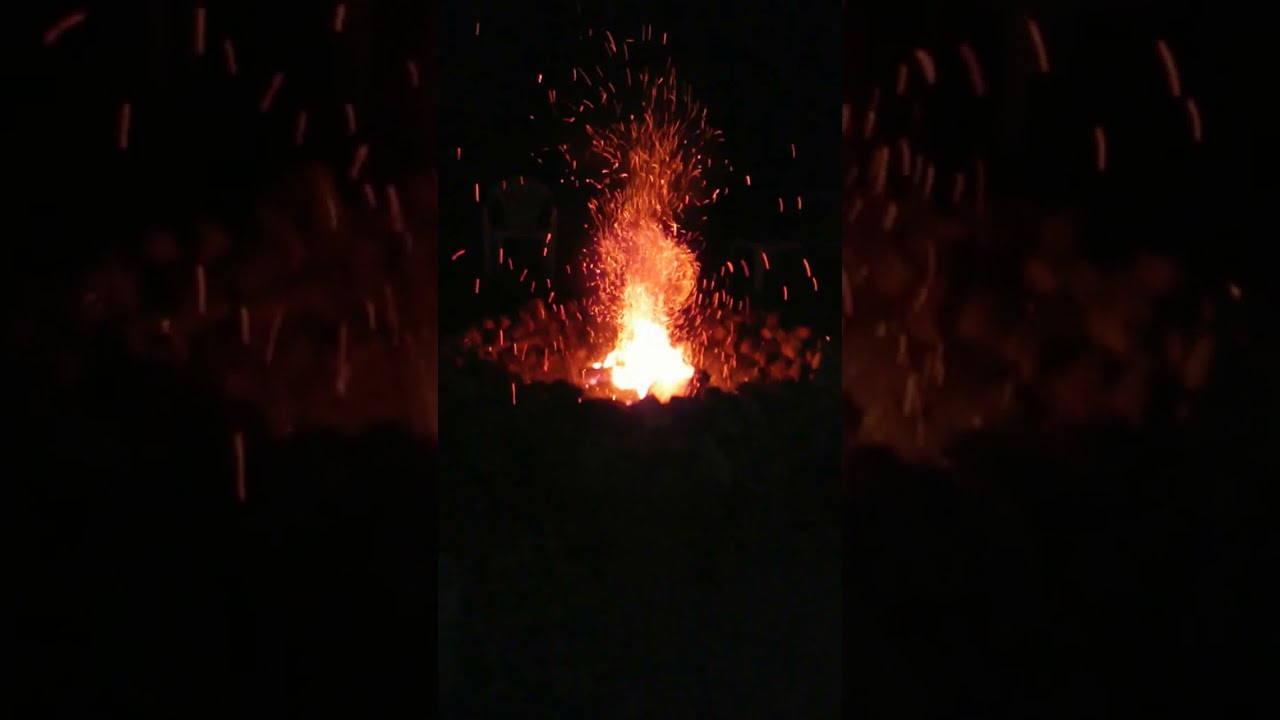This photograph captures a vividly intense and simple scene, dominated by a central, fiery composition. The entire backdrop of the image is engulfed in blackness, enhancing the stark contrast with the bright, white-hot to red-hot flames at the center. The fire, possibly from a cauldron or crucible, radiates an eerie glow, illuminating its immediate surroundings. Numerous sparks crackle and swirl upwards from the intense flames, creating dynamic patterns of light against the dark background. The fire itself exhibits rich hues of yellow, orange, and red, suggesting either a combusting material or molten metal being poured. Beneath the flames, there appear to be rocks or coals fueling the blaze. This outdoor scene lacks any visible text or figures, emphasizing the raw and powerful nature of the fire and its sparks, which seem to leap out energetically into the night.